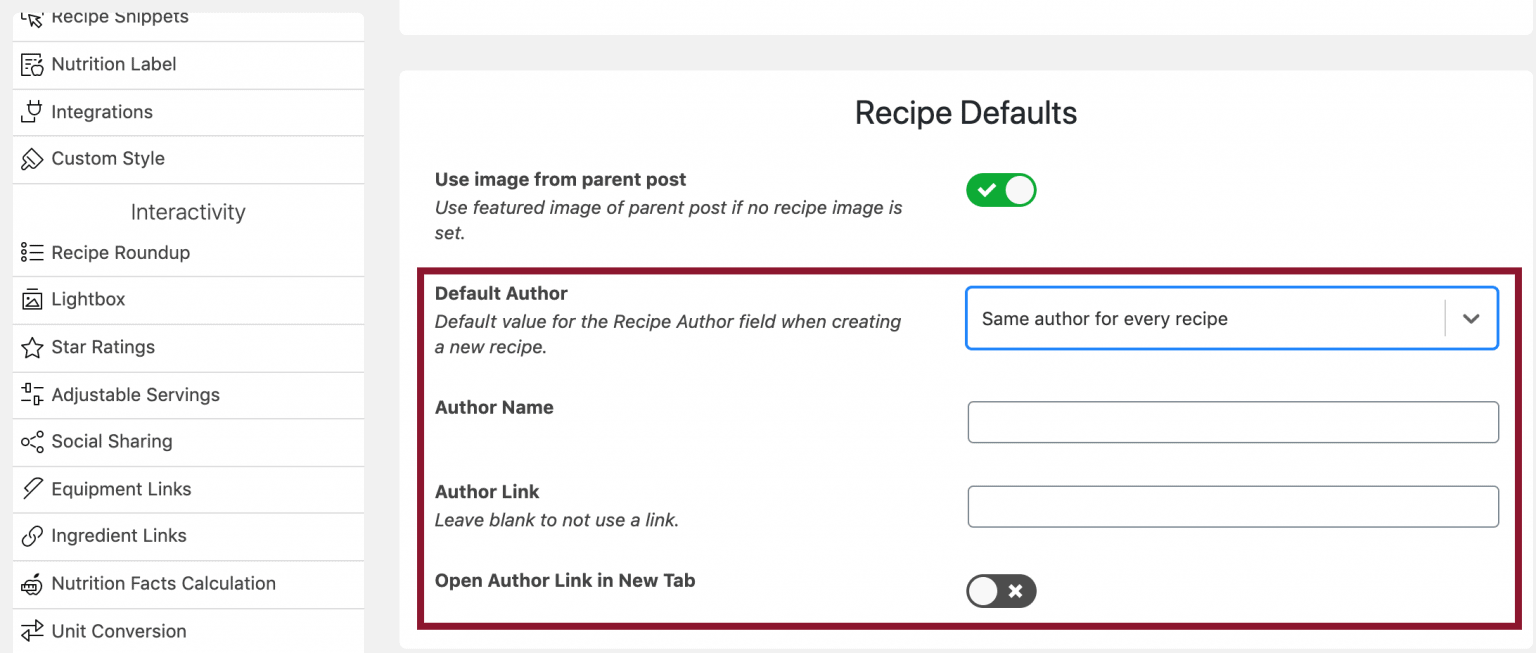Here is a cleaned-up and detailed caption based on the provided description:

---

The page is divided into two sections, each framed with a gray outline and containing various elements. 

**Left Section:**
This section is titled "Recipe Snippets" in black text, with the top part slightly cut off. The background is white with several thin gray horizontal lines creating rows. Each row contains text labels in gray, as follows:
- Nutrition Label
- Integration
- Custom Style
- Inactivity Recipe Rounded-Up
- Light Box
- Storage
- Adjustable Service
- Social Sharing
- Equipment Links
- Ingredient Links
- Nutritional Facts Calculation
- Unit Correction

**Right Section:**
This section is titled "Recipe Defaults" in black. The background features a dark red border. Inside, under the header "Use Image From Parent By Default," it states: "Use feature image of parent post if no recipe image is set." Below this, the section describes the "Default Author" settings:
- "Default author" specifies the default value for the recipe author field when creating a new recipe.
- A white input box outlined in blue follows, with the text "Same author for every recipe" above it.
- "Author Name," followed by an empty input box.
- "Author Link," with instructions to leave blank to not use a link, followed by another empty input box.
- At the bottom, there is a checkbox option "Open author link in new tab," followed by a gray oval switch with a white circle on one side and a gray 'X' on the other side.

---

This detailed description captures both the structure and the specific content of the image, providing a clear understanding of the layout and elements within each section.